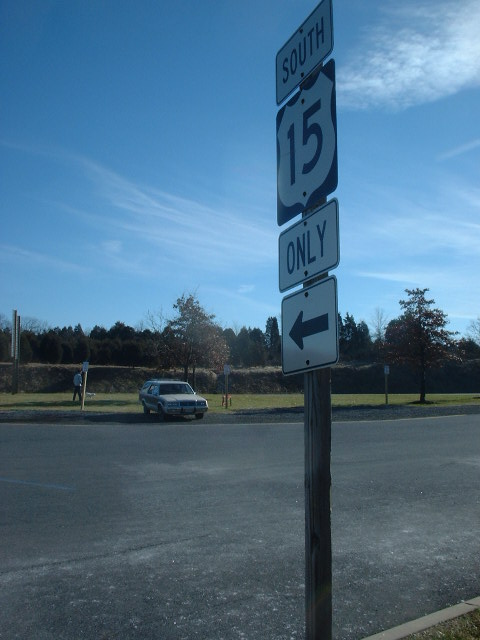This photograph captures a roadway scene featuring a prominently displayed highway sign on square wooden posts. The sign is composed of four distinct parts: a white rectangular sign at the top labeled "South," directly beneath it a white shield-shaped sign with the number "15" in black text, followed by another white rectangular sign with the word "only" in black text, and finally, a black arrow pointing to the left. 

In the foreground, notably positioned is a single car parked adjacent to the concrete road. A man is seen walking near the car, adding a sense of liveliness to the scene. The background reveals a serene, almost clear blue sky dotted with sparse white clouds, a patch of green grass possibly suggesting a field, and a dense forest of trees. Another sign can be seen in the image, although it appears to contain no discernible text. This thriving greenery and expansive sky provide a peaceful backdrop to the otherwise functional and directive nature of the road sign.